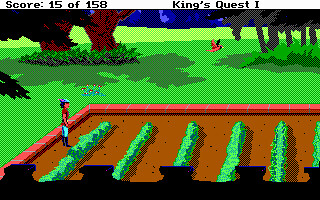This is a screenshot from the computer game "King's Quest 1" showing a cleared area surrounded by masonry walls. At the top of the image, the game displays the score as 15 out of 158. On the left side of the scene stands a man dressed in boots, blue pants, a red top, and a blue hat. The area is adorned with neatly arranged rows of light green hedges or vegetation, each shaded on the right side. At the forefront of the image, five black parapets can be seen, each with a hint of blue on their tops, giving a fortified appearance. In the background, a wooded area with sparsely growing trees and green grass can be observed, with the sun casting shadows on the ground beneath them. Adding a touch of life to the scene, a bird is captured mid-flight in the center-left of the image. The predominant color throughout the background is green, contributing to the lush and vibrant atmosphere of the setting.